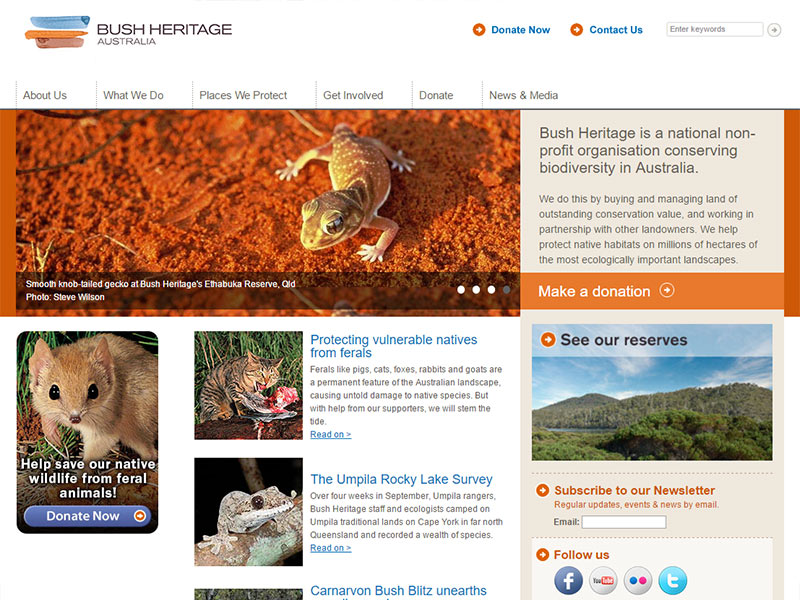This screenshot captures a cropped section of a white-background web page belonging to Bush Heritage Australia. Prominently at the top left is the Bush Heritage Australia logo. Adjacent to it on the right are two small, blue, bold options: "Donate Now" and "Contact Us." Each is prefaced by an orange circle with a right-pointing arrow. Further right is a small text box labeled "Enter Keywords."

Below the header, a horizontally arranged list of categories spans the page in gray font: "About Us," "What We Do," "Places We Protect," "Get Involved," "Donate," and "News and Media." Beneath this menu, a large rectangular image of a gecko is displayed. Overlaid on the lower part of the image is a semi-transparent black box featuring the name of the animal on the left and the photographer's credit. To the right side of this overlay, four dots suggest that this is the third image in a sequence of four, which users can navigate by clicking the dots.

To the right of the gecko image, a gray box contains a description of Bush Heritage. Directly below this informational section is a prominent orange bar with the text "Make a Donation." This bar includes a white circle outline with a white arrow inside, indicating that clicking it will redirect the user to the donation page.